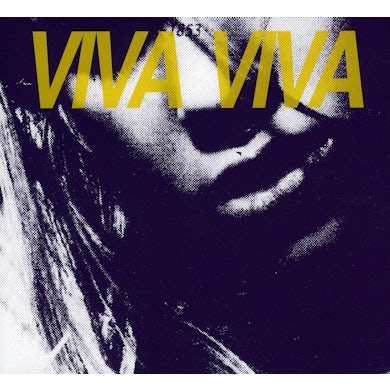The image resembles a black-and-white photograph with a digital filter, giving it a slightly pixelated effect. It prominently features the lower half of a woman's face, highlighting her mouth, nose, and some of her hair, with the rest of her face obscured by shadows. The visible parts of her face are illuminated in white against a navy background, giving it a rainy, contemplative appearance. At the top center of the image, large yellow capital letters spell out "VIVA VIVA." In small black print above the text, the digits "1853" are displayed, suggesting a vintage or historical theme.